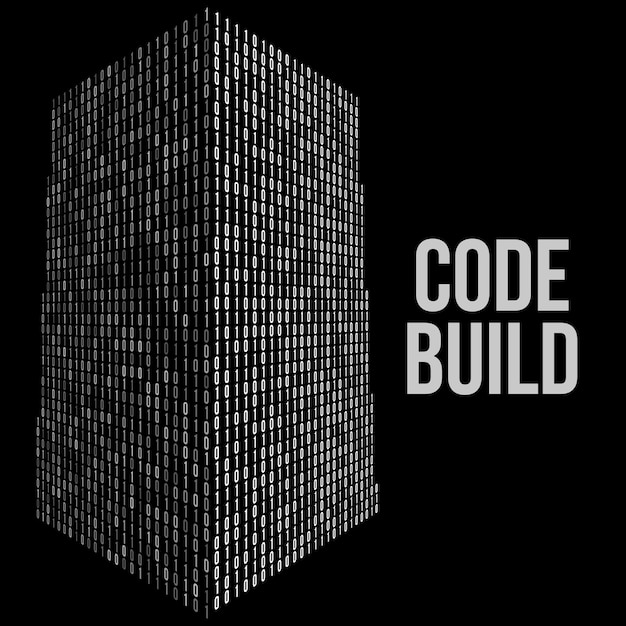The image portrays an advertisement-like flyer with a stark black background. On the right side, bold and all-uppercase letters spell out "CODE BUILD" in a sleek, white or gray printed font. Dominating the left side is a distinctive 3D structure, reminiscent of a tall building viewed from an angular perspective. This geometric shape is meticulously constructed from an array of 1’s and 0’s, creating a compelling visual of a binary-coded edifice. The numbers are uniformly gray, and the structure's design suggests depth, making it appear like a complex, data-driven monolith emerging from the dark background. There are no other colors or objects present in the image, focusing attention solely on the textual and numeric elements.